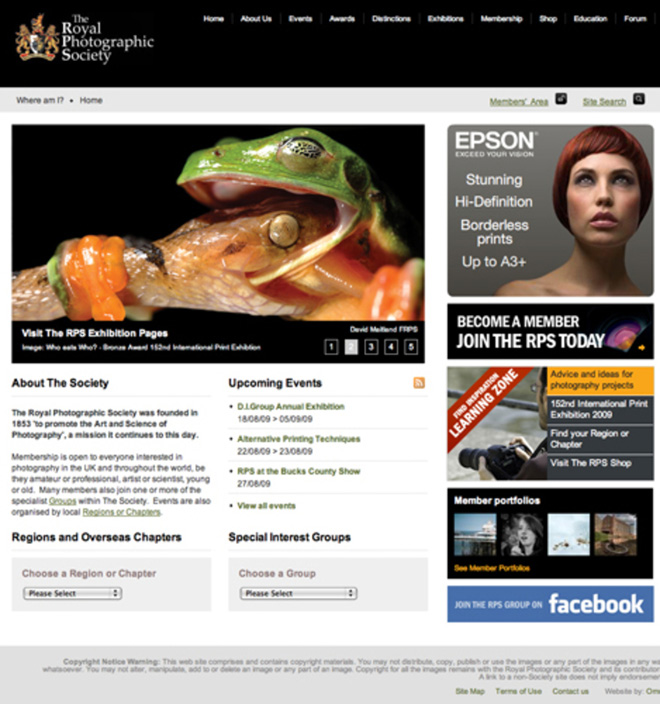This image, captured from a computer screen, prominently displays a webpage of the Royal Photographic Society (RPS). Centrally featured is a striking photograph of a snake consuming another snake, with the prey’s head partially inside the predator’s mouth, showcasing an intense moment in nature. Above the image, a headline encourages visitors to explore the RPS exhibition pages.

Below the photograph, detailed text describes the society’s rich history and mission. Founded in 1853, the Royal Photographic Society aims to promote the art and science of photography, a goal it continues to uphold. The text highlights that membership is open to anyone interested in photography, whether they are amateurs, professionals, artists, or scientists, irrespective of age. It notes that many members also join one or more of the specialized groups within the society. Moreover, local regions or international chapters organize various events, reflecting the society’s global reach.

On the right-hand side of the screen, a series of advertisements are visible, including promotions for Epson and Facebook among other sponsors. Additional sections of the webpage mention information about the society, upcoming events, and special interest groups, offering a comprehensive overview of the RPS and its activities.

The overall image provides an in-depth glimpse into the Royal Photographic Society's online presence, emphasizing its century-long dedication to the photographic community.